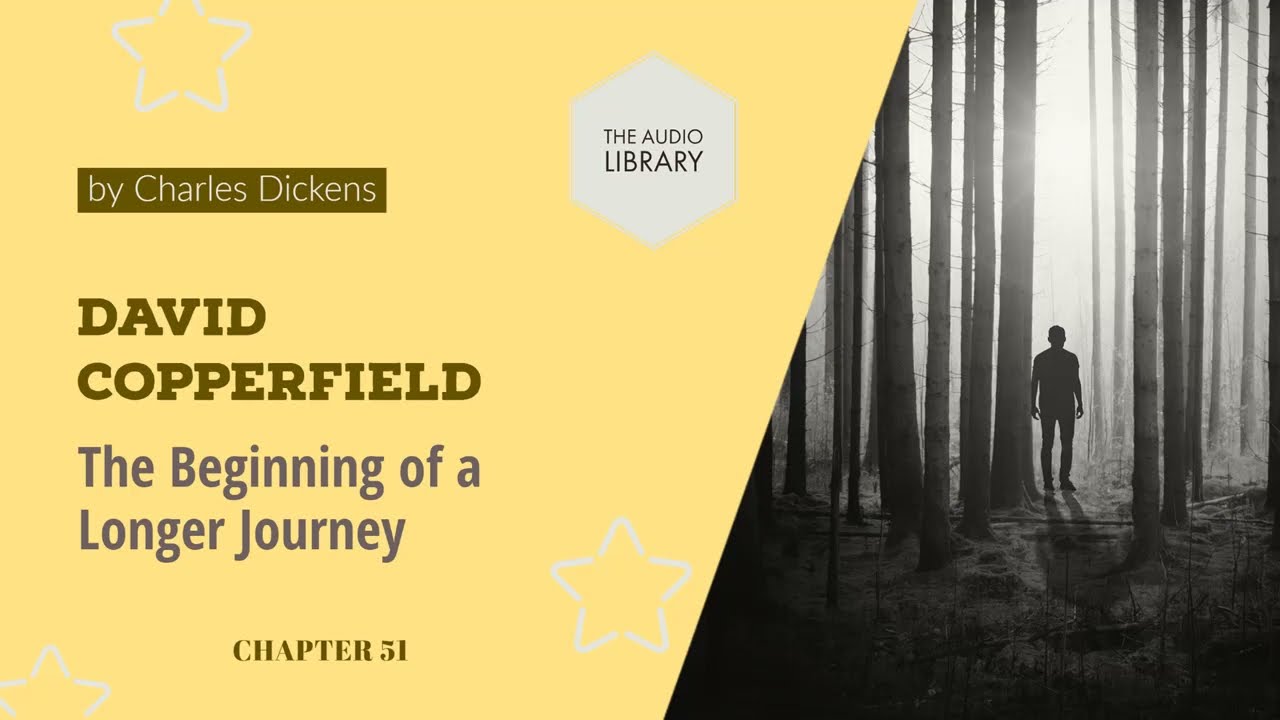This image is an advertisement for an audiobook, featuring a visually striking design divided into two main sections. The left side of the rectangular poster has a yellow background adorned with a few small white star outlines. At the top of this yellow section, a white hexagon or diamond-shaped icon contains the text "The Audio Library." Directly below this, a black rectangle showcases the author's name, "by Charles Dickens," followed by the title, "David Copperfield." Further down, in blue letters, it reads, "The Beginning of a Longer Journey," and beneath this is the label "Chapter 51."

The right side of the poster contrasts sharply with a black-and-white photograph showing a man silhouetted against a nighttime forest scene. He stands among thin, tall tree trunks rising from a dirt-covered ground. The man’s features and attire are obscured due to the silhouette effect created by the light source. The overall aesthetic combines the evocative imagery of the monochrome forest with the informational text on the bright yellow background, effectively promoting the audiobook.